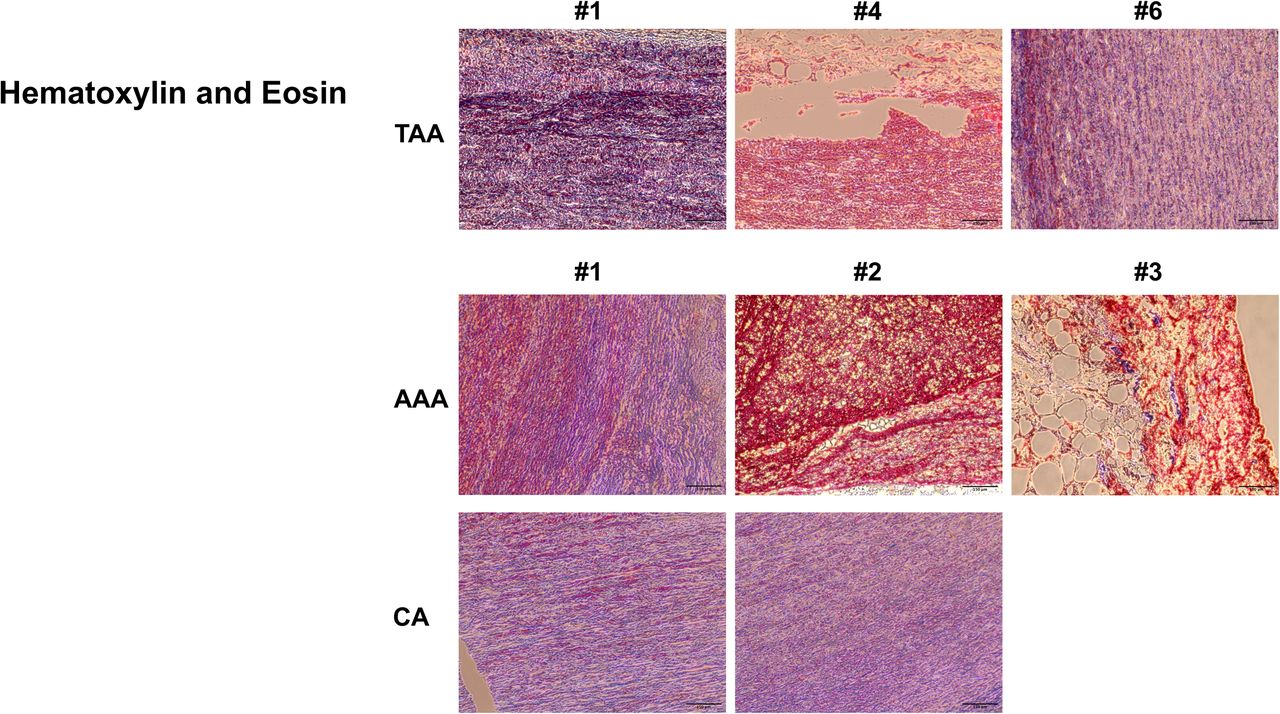This image is a detailed scientific illustration showing a grid of microscopic slide photographs stained with hematoxylin and eosin. The grid is organized into three rows: the first row, labeled "TAA," contains three pictures numbered 1, 4, and 6; the second row, labeled "AAA," also contains three pictures numbered 1, 2, and 3; and the third row labeled "CA," contains two pictures. The labels are positioned along the top and left sides of the grid. The slides display vivid colors including shades of purple, fuchsia, red, beige, and pink, and reveal detailed textures of what appears to be cell or skin tissue. The large black text on the left reads "hematoxylin and eosin," emphasizing the staining technique used in these exceptionally sharp, close-up scientific photographs.